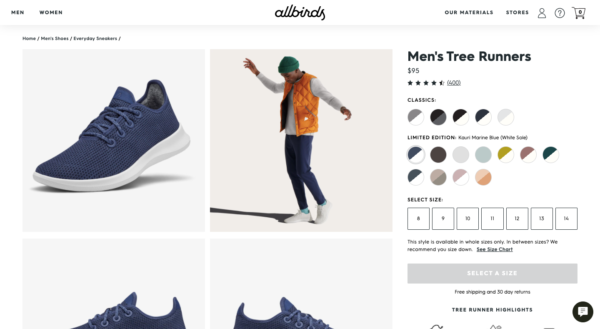The webpage for "All Birds" features a clean, white background with the title elegantly displayed at the top in cursive text. In the upper-left corner, two navigation options labeled "Men" and "Women" stand out in black font. Centrally positioned are four images, with only the top two fully visible while the bottom two are partially cut off.

The top-left image showcases a sleek blue shoe with a white sole, oriented to the left. Next to it, a photograph features a stylish black man dressed in a long-sleeved gray shirt and an orange vest. He is wearing jeans, gazing down at his white shoes, and posing with arms outstretched, facing left. His shadow extends to his left.

The bottom-left and bottom-right images provide close-up profiles of the blue shoe, focusing on the lip and shoelaces, although only their tops are visible.

On the right side of the webpage, a detailed product description reads: "Men's Tree Runners, $95." The product boasts a rating of four and a half stars out of five, based on 400 reviews. Numerous color options are presented in circles, each divided diagonally into two colors. Combinations include gray-white, black-gray, black-white, blue-white, among others. 

Two categories of options are available: "Classics" with five color choices, and "Limited Edition" offering 11 different options. Below the color options, there's a "Select Size" section featuring sizes in both standard (XS, S, M, L) and numerical formats (8, 9, 10, 11, 12, 13, 14).